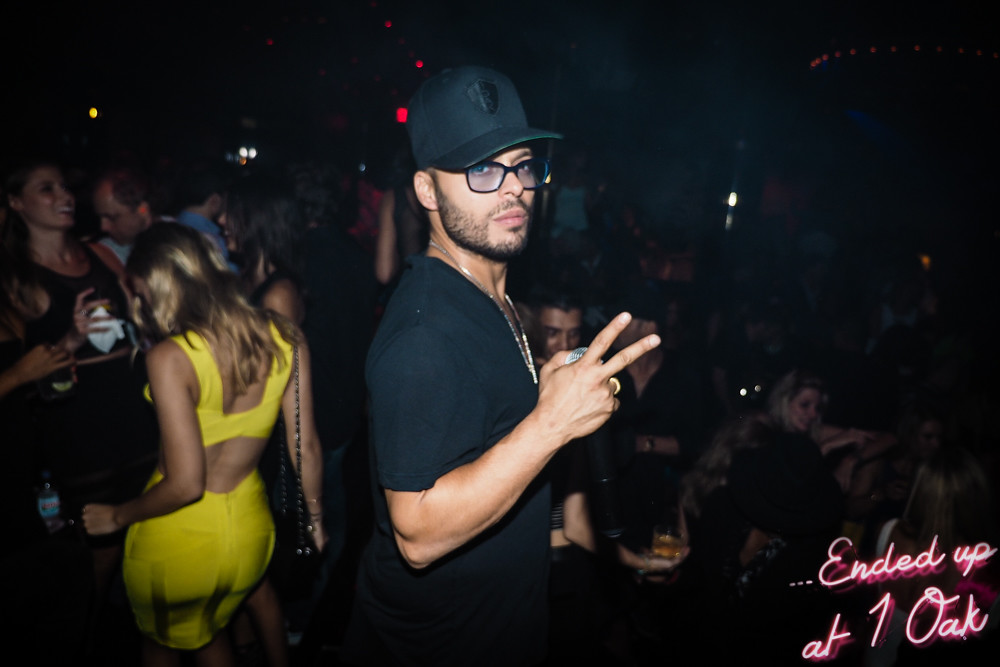The image captures a lively scene that appears to be set in a club or bar, featuring a man as the central figure. The man is wearing a black baseball cap, black-rimmed glasses, a dark grey t-shirt, and a medal around his neck. He sports a mustache and slight beard. Positioned to the side, he looks back at the camera, raising his right hand to display a peace sign while holding an object in his other hand.

To his left and behind him stands a woman who particularly stands out. She is dressed in a yellow outfit that includes a bra top and a tight skirt that reaches just above her knees. The outfit is notable for its back cut-outs along her shoulders and lower back. She has long blonde hair that falls to mid-back, and she is turned away from the camera, revealing her bare arms.

In the background, the club is bustling with various other patrons who appear to be either seated around tables or standing, engaged in conversation and enjoying the ambiance. A woman in a black sleeveless jersey and a man wearing a blue shirt can be seen among the crowd.

The lower right corner of the image features a red glowy text with shading, designed to resemble a neon sign, which reads, "Ended up at One Oak." The text adds to the visual vibrancy of the scene, contrasting with the dark, lively atmosphere of the club.